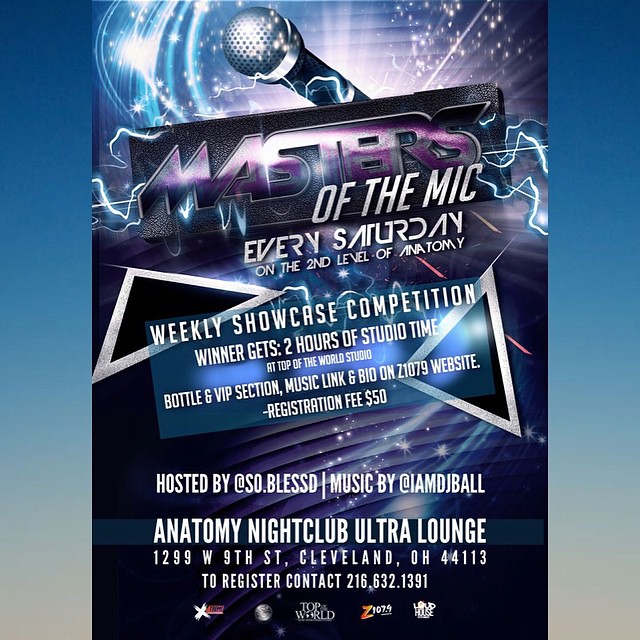This vertically aligned rectangular advertisement features a vivid blue background at the top, transitioning gradually to white at the bottom. The centerpiece is another vertical rectangle showcasing a vibrant galaxy theme with swirling stars. Dominating the upper section is an image of a silver and black microphone adorned with glitter, lightning bolts striking down its length. At the top, block letters spell out "MASTERS" in illuminated purple with white accents, followed by "OF THE MIC" in bold white capital letters.

The design announces "Masters of the Mic" held every Saturday on the second level of the Anatomy Nightclub Ultra Lounge. Midway down, a diagonal rectangle proclaims the "Weekly Showcase Competition," with enticing details such as a two-hour studio time prize at Top of the World Studio, a bottle service in VIP, and a music link provided on the Z1079 website. The registration fee is set at $50. Along the bottom, it mentions that the event is hosted by @so.blessed and features music by @imdjball. The venue is clearly indicated as Anatomy Nightclub Ultra Lounge, 1299 West 9th Street, Cleveland, Ohio 44113, with contact details for registration provided: 216-632-1391.